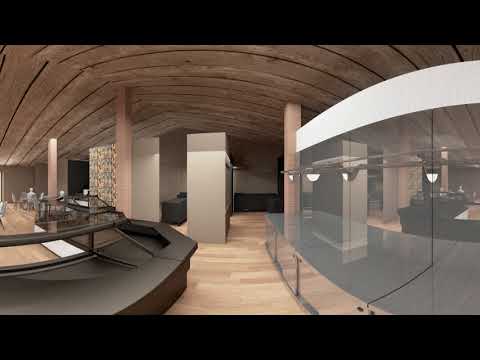The photograph depicts a spacious, well-lit indoor room, possibly a restaurant or an office building. The room features an architecturally striking curved ceiling made of dark wood and a light wood-paneled floor, creating a warm and inviting atmosphere. Prominent square, dark tan pillars support the ceiling at various points throughout the space.

On the right side of the image, there is a large reflective glass partition wall. Inside the glass, several lamps are installed, suggesting that this section of the room is still under construction or being prepared for an intricate display. Additionally, there is a smaller display case or counter area with a brown base and a black top, equipped with empty frames likely meant for holding descriptive information once fully set up.

In the background, rows of shelving or library stacks are visible, adding a sense of organization or storage capability to the room. Towards the far left corner, a solitary person is seated at a table, lending a touch of activity to the otherwise pristine and spacious environment. A long counter with a glass display case is positioned along this side, empty but ready to showcase items in the future. Overall, the photo captures an elaborate, thoughtfully designed space, blending wood and glass elements harmoniously.